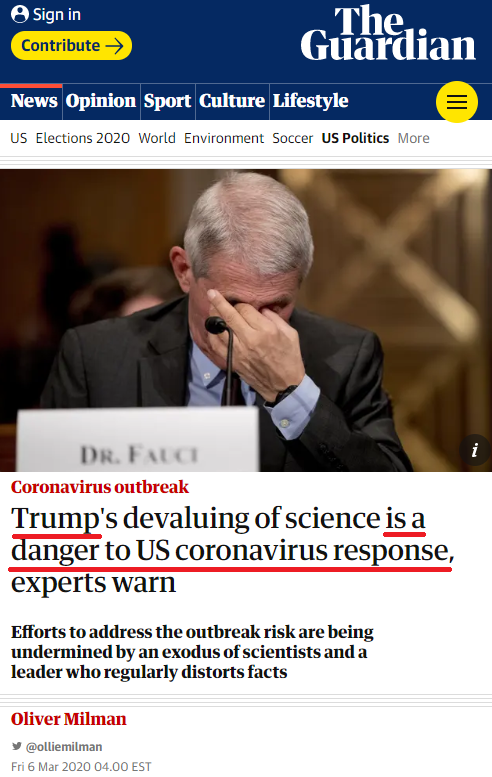This image is a screenshot of a smartphone displaying a section of The Guardian's website. At the very top, there's a dark blue band with the word "Sign in" written in blue text. Below that, on a yellow band background, the word "Contribute" is displayed in blue with a right arrow symbol next to it. The title "The Guardian" is prominently showcased in white text beneath these elements.

Following the title, there's a navigation menu that includes options such as "News," "Opinion," "Sport," "Culture," and "Lifestyle." Below this menu, the section headline "U.S. Politics" is featured.

In the central portion of the image, there's a picture of a man covering his eyes with his hand. The article headline below the picture reads "Dr. [Name withheld] says coronavirus outbreak," with "coronavirus outbreak" highlighted in red ink. Below the headline, there is another significant phrase underlined in red: "Trump's devaluating of science as a danger to U.S. coronavirus response." The rest of the text appears to be body content in standard black ink. 

This section of the website is dedicated to a news piece focusing on U.S. politics and the coronavirus outbreak, specifically concerning the implications of undermining scientific advice in the context of the pandemic response.